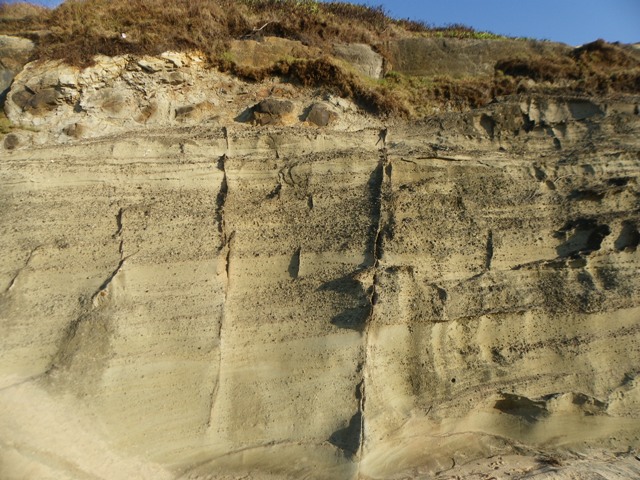The image depicts a striking photograph of a steep, bright brown cliff face, resembling a canyon. At the base, a sandy floor is visible, characterized by scattered boulders and rocks. The cliff walls exhibit intricate patterns likely formed by wind erosion, adding texture to the vertical expanse. Near the top, patches of green and brown dry bushes and shrubs can be seen, indicating a mix of surviving and desiccated vegetation. Above the cliff, a sliver of bright blue sky is visible, contributing to the arid atmosphere of the scene. Scattered throughout the image are subtle hues of tan, gray, and even black, portraying the complex interplay of natural elements in this rugged landscape.